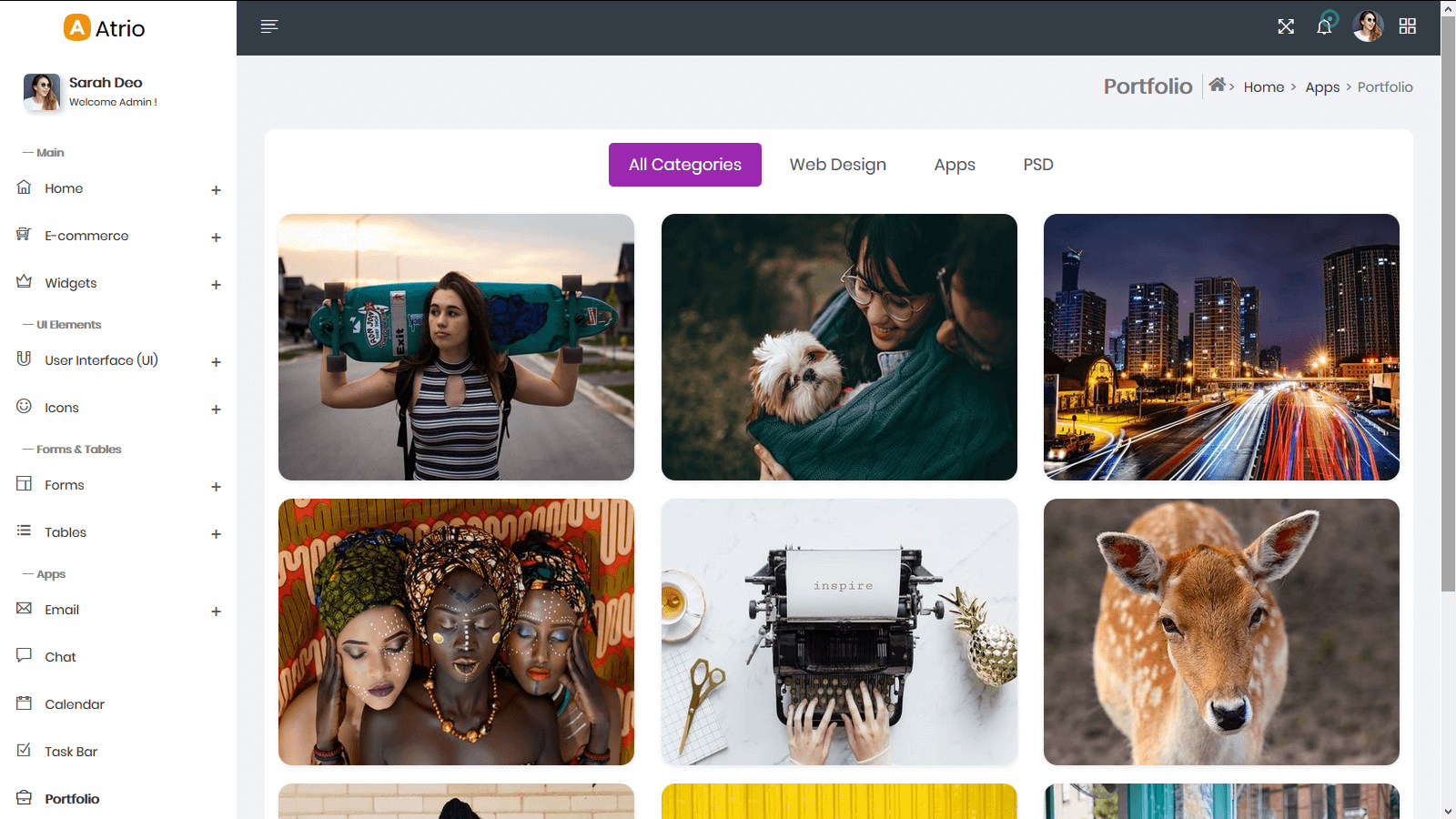The image appears to be a screenshot from a website called Atrio, evident from the label "Atrio" positioned in the top left corner. Accompanying this label is a stylized 'A' set within a yellow oval. Below, there is a white section filled with black text, prominently welcoming the user, "Sarah Dio," with a message stating "Welcome Admin." Adjacent to this greeting is a small square photograph of a white woman with long hair and sunglasses.

The website features a navigational menu listing several clickable options, including Home, E-commerce, Widgets, User Interface, Icons, Forms, Tables, Email, and Chat. To the right side of the screen, there is a rectangular area displaying a collection of images. This section appears to be sorted under "All Categories," denoted by a blue rectangle bearing white text at the top.

The visual content within this area comprises six distinct pictures:
1. At the top left, a woman with long, dark hair, clad in a gray and black striped tank top, is seen walking down a road with a skateboard slung over her shoulders.
2. To the right of this, an individual with dark hair and glasses is pictured holding a dog.
3. The upper right section showcases a vibrant nighttime city scene, highlighted by the streaking lights of cars in motion.
4. In the lower left, three women are depicted with their eyes closed, heads gently resting against each other to convey a sense of peace.
5. Centrally located at the bottom, someone is captured typing on an old-fashioned typewriter.
6. Lastly, the bottom right corner features a close-up image of a brown and white deer facing the camera.